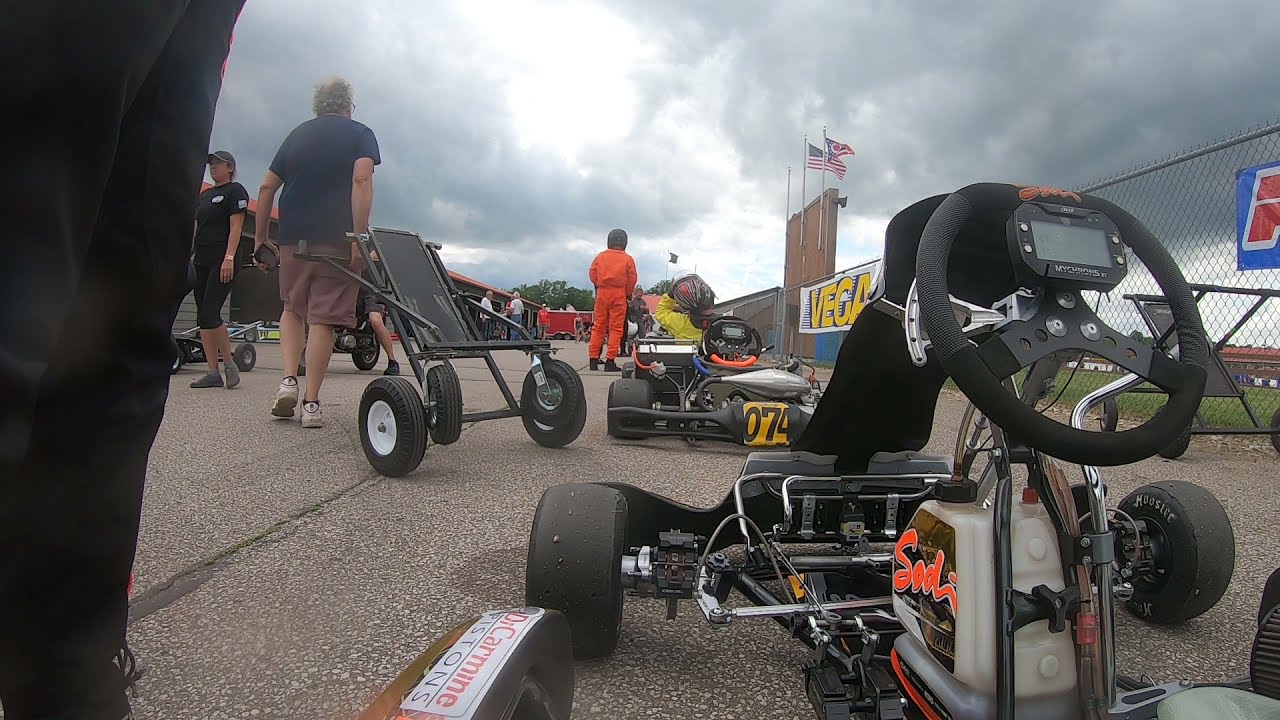In this outdoor scene, the image captures the bustling preparations for a go-kart race. The foreground prominently features a close-up of a go-kart, showcasing its large black steering wheel equipped with an instrument panel and a digital display. The go-kart's gas tank is tucked beneath the steering wheel, and its wide front tires are clearly visible. Just ahead, another go-kart sports a yellow banner with the black number 074. Adorning the side of the first go-kart are the orange letters "S-O-D-I."

Among the crowd, a man in a dark blue t-shirt and burgundy shorts is seen pulling a metal wheeled cart, while another person in an orange jumpsuit with a helmet stands in front of the second go-kart, likely one of the drivers. Another man in a short-sleeved blue shirt and khaki shorts is situated to the upper left, next to someone in a black t-shirt and shorts. 

Flanking the scene, a chain-link fence hosts several banners, with an American flag flying near the race area. The backdrop includes a building with more flags visible above it and some grass behind the fence. Dominating the upper portion of the image, the sky is overcast with large gray clouds, adding a dramatic tone to the scene filled with anticipation and excitement.